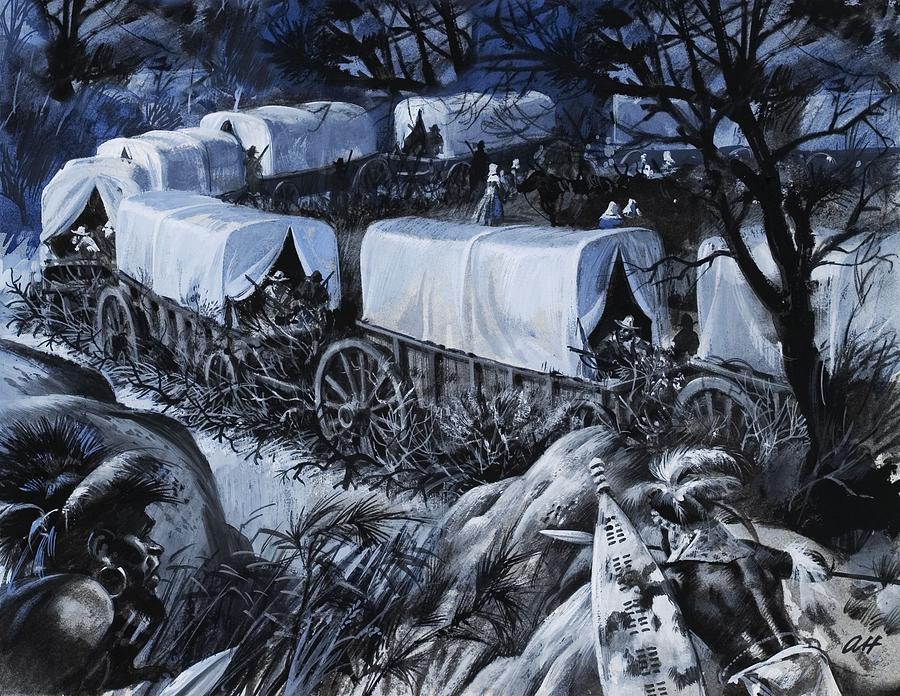The artwork, featuring a signature in the corner in black ink, showcases an almost illustrative quality rendered in tones of blues, whites, and blacks. The foreground presents two Aboriginal men, both crouching behind some rocks amidst overgrown grass. One man, adorned with a feathered headdress, clutches a spear, while the second, also wearing a feathered headdress and a distinctive earring, has black facial hair.

In the scene's midground, a caravan of covered wagons stretches across the landscape, their white coverings vibrant against the muted tones of the image. Figures equipped with shotguns accompany the wagons, while women in long dresses and head coverings mill about, adding to the bustle of the scene. Leafless trees and overgrown brush dot the background, adding a sense of rugged wilderness to the composition. This dynamic tableau depicts the caravan moving right past the hiding men, fusing elements of suspense and everyday life into a compelling narrative moment.